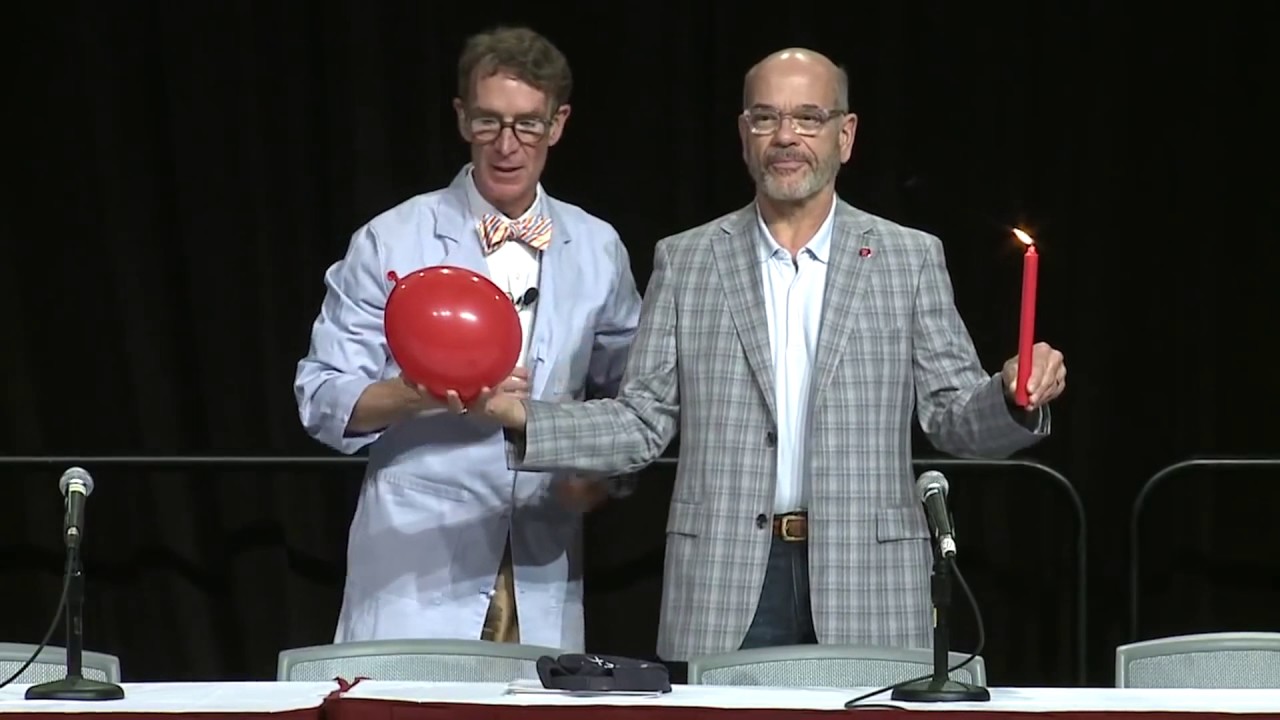The photograph captures Bill Nye the Science Guy on the left, recognizable in his iconic outfit featuring a baby blue lab coat, a bow tie, and his characteristic thick glasses. He has medium-length brown hair and is looking intently down at an inflated red balloon, his mouth open as if he is in the middle of explaining something. To the right stands a bald man with a greying well-trimmed beard, wearing glasses and a grey plaid overcoat with a white button-down shirt underneath. In his left hand, he holds a lit red candle, the flame visible, and in his right hand, stretched out in front of Bill Nye, he holds the red balloon. They are both standing behind a banquet table equipped with two microphones and several chairs, all set against a solid black background, suggesting a presentation or demonstration scene.